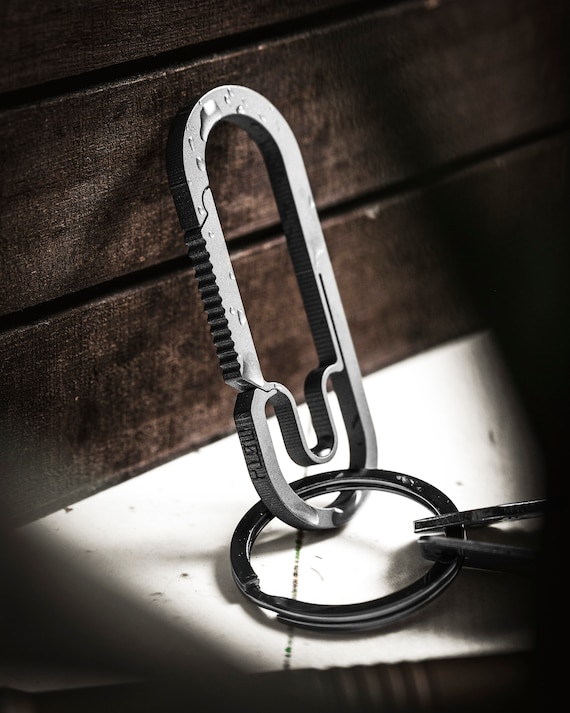This vertical rectangular image showcases a dark-stained wooden wall composed of horizontal slats. Affixed to this wall, possibly resting against a small, white painted wooden shelf or surface, is a sizeable, silver oval-shaped key ring with grooved edges and some water spots on it. There are initials inscribed on the key ring, adding a personalized touch. Attached to the key ring is a circular metal ring, also silver, which lies flat against the white surface. Across the key ring, positioned on top of the circular ring, are the tips of what appear to be a pair of pliers or tweezers. The lower left corner and parts of the middle and right side of the white surface are cast in shadow.